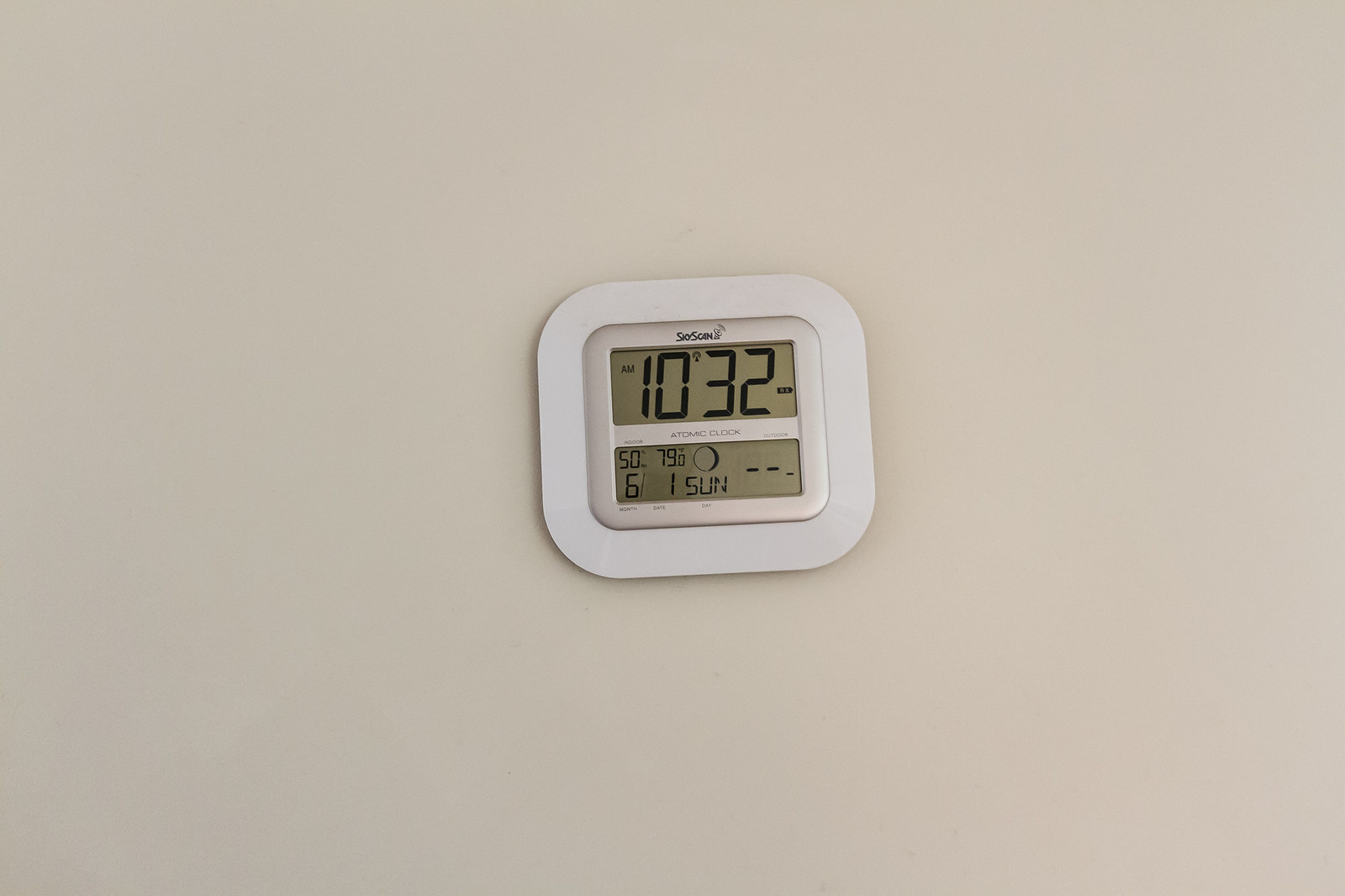This indoor photograph features a thermostat mounted on an eggshell white wall, subtly illuminated by natural daylight, suggesting it was taken during the daytime. Centered in the image, the thermostat is slightly tilted to the left, emphasizing its square shape with rounded corners and a white frame. Prominently displayed in black font is the "SkyScan" logo accompanied by a satellite icon. The digital clock on the thermostat shows the time as 10:32 AM. Below the clock, a separate screen indicates the indoor temperature as 50 degrees, while 79 degrees is displayed to the right, possibly denoting the outdoor temperature or a set temperature. The date is shown as June 1st, and it is identified as a Sunday. "Atomic Clock" is inscribed between the two screens, and an icon illustrating the moon is located above the day of the week.